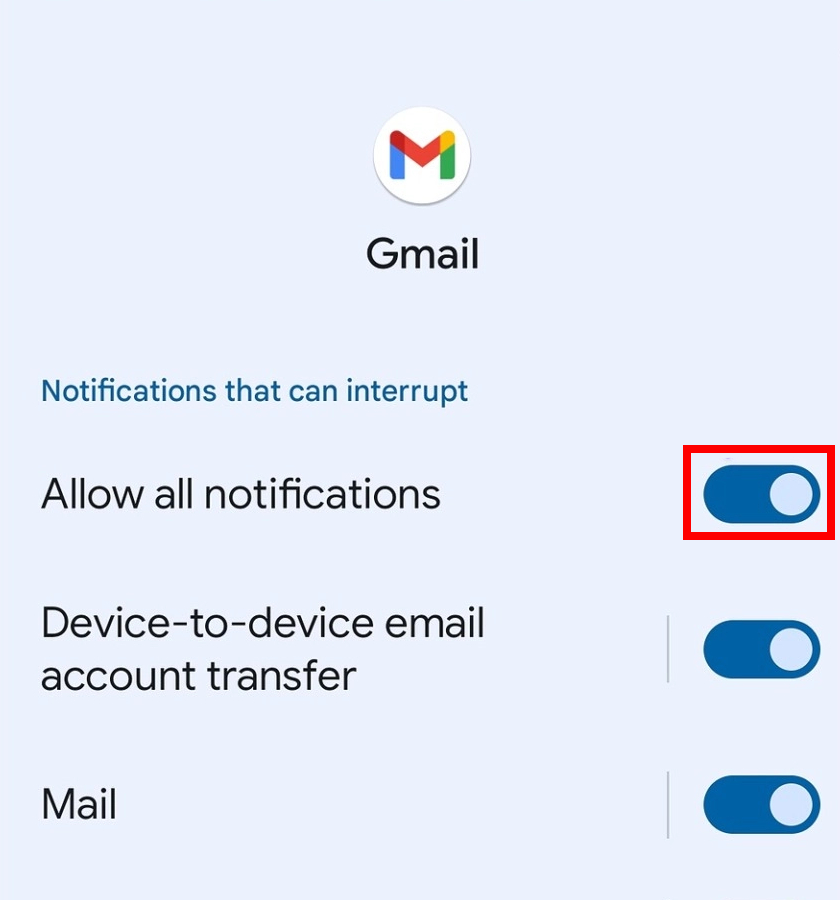The screenshot displays a section of the Gmail app interface focused on notification settings. At the top center of the image, the Gmail logo is prominently displayed with the word "Gmail" right below it. Directly underneath, a blue-highlighted header reads "Notifications that can interrupt," indicating the settings are related to managing interruptions from notifications.

There are three main notification options shown in black text, each accompanied by a toggle button to the right:

1. "Allow all notifications" - This option is emphasized with a red rectangle surrounding the toggle button, which is currently turned on.
2. "Device to device email account transfer" - Shown in black lettering with its corresponding toggle button also turned on to the right.
3. "Mail" - Also displayed in black text with the toggle button to the right, which is turned on as well.

The background of the settings interface is off-white, and all the toggle buttons exhibit a blue color, indicating they are active. This screen is evidently a part of the Gmail app's settings where users can enable notifications that might interrupt their activities, such as phone calls or other tasks.